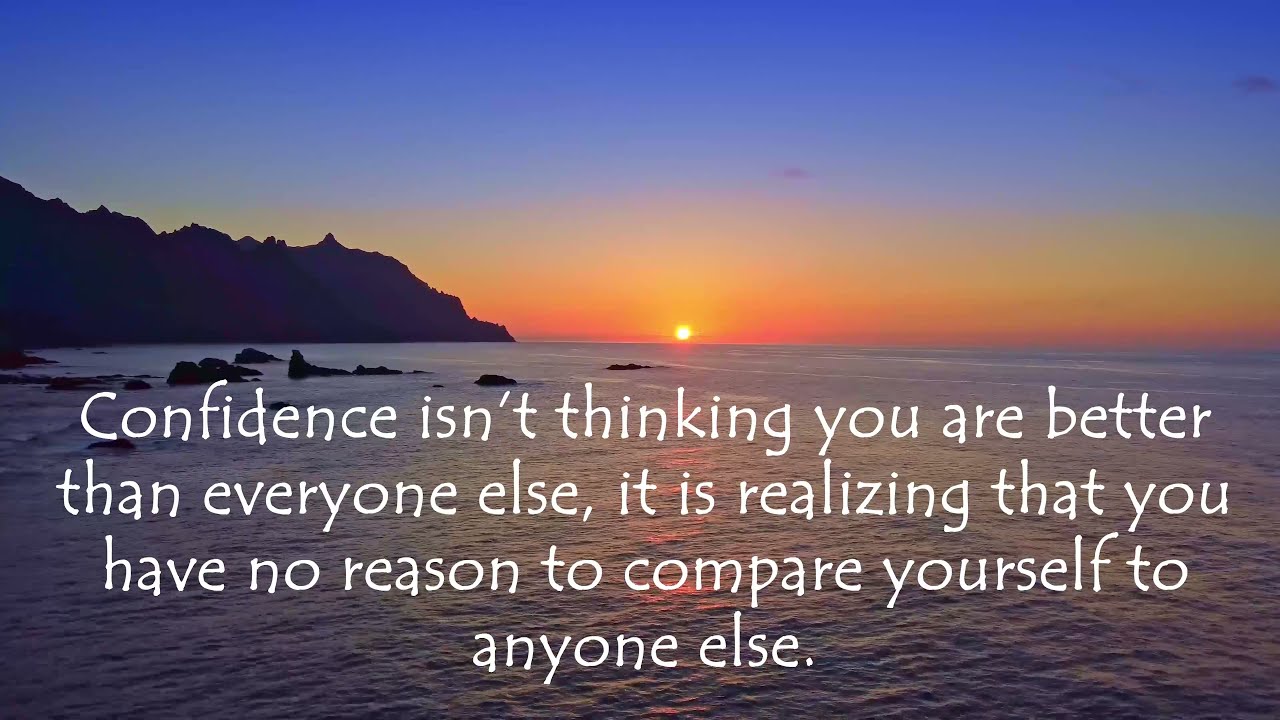The image is a color photograph of a serene ocean at sunset. The bottom half of the image showcases the calm blue ocean, while a rocky outcropping extends from the left edge almost to the center. This promontory of land features hills and rocks jutting out into the water. In the background, a deep yellow sun touches the horizon, casting hues of pink, gold, and orange across the sky, which gradually transitions to deep blue at the top. Overlaid in white print across the ocean is an inspirational message that reads: "Confidence isn't thinking you are better than everyone else, it is realizing that you have no reason to compare yourself to anyone else." The text is center-aligned, with the last line positioned just beneath the sun, highlighting the image's central focal point.